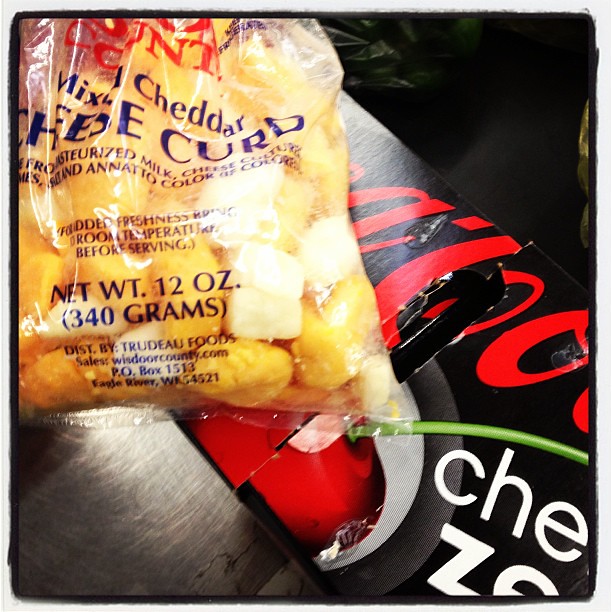The photograph captures a detailed scene of a food product setup on a stainless steel table. Anchored in the upper left corner is a bag of mixed cheddar cheese curds, conspicuously displaying its label which states a net weight of 12 ounces (340 grams) and identifies the distributor as Trudeau Foods, located at P.O. Box 1513, Eagle River, WA 54521. The cheese curds inside the partially visible bag reveal a blend of yellow and white pieces. In the backdrop, there is a prominent cherry-flavored Coca-Cola Zero box, suggestive of a 24-pack, characterized by its red text on a black background. This box shows clear signs of prior handling, evidenced by the finger pull tabs. The overall composition suggests that the image was taken from a high angle, looking down at the metallic table, capturing just enough to give context without revealing the entire setup or product details fully.